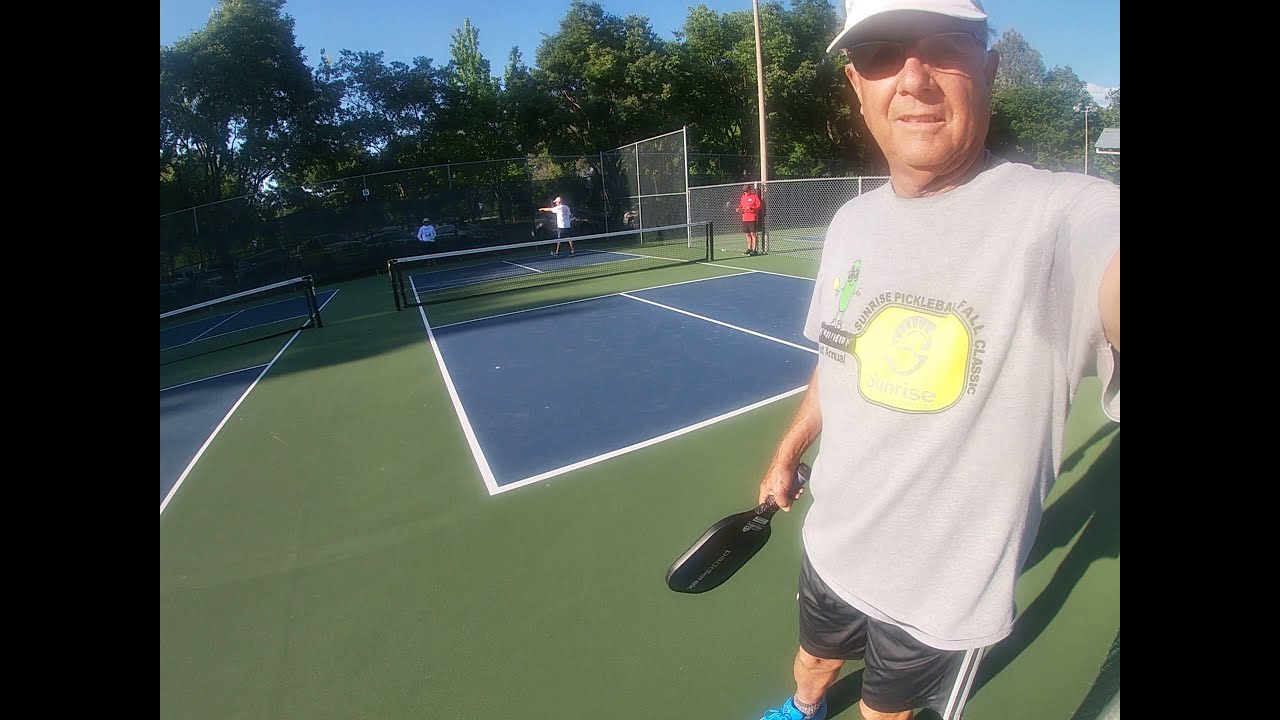In this full-color, landscape-oriented photograph taken on a sunny day with a clear blue sky and no clouds, an older gentleman, likely in his early to mid-60s, is featured taking a selfie in the foreground. He is standing on a pickleball court, distinguishable by its dark green surroundings, blue playing area, and white outlines. The man, sporting a white brim cap and sunglasses, wears a gray shirt with a yellow graphic associated with a pickleball league or event and has visible sweat stains under his arms. He also wears black shorts and blue shoes. Holding a pickleball racket in his right hand by his side, he smiles at the camera. In the background, a few other men are either waiting or engaged in a game, partially visible through the shade cast by surrounding trees. The image captures the essence of a fun day outdoors, playing pickleball under the vibrant, clear skies.